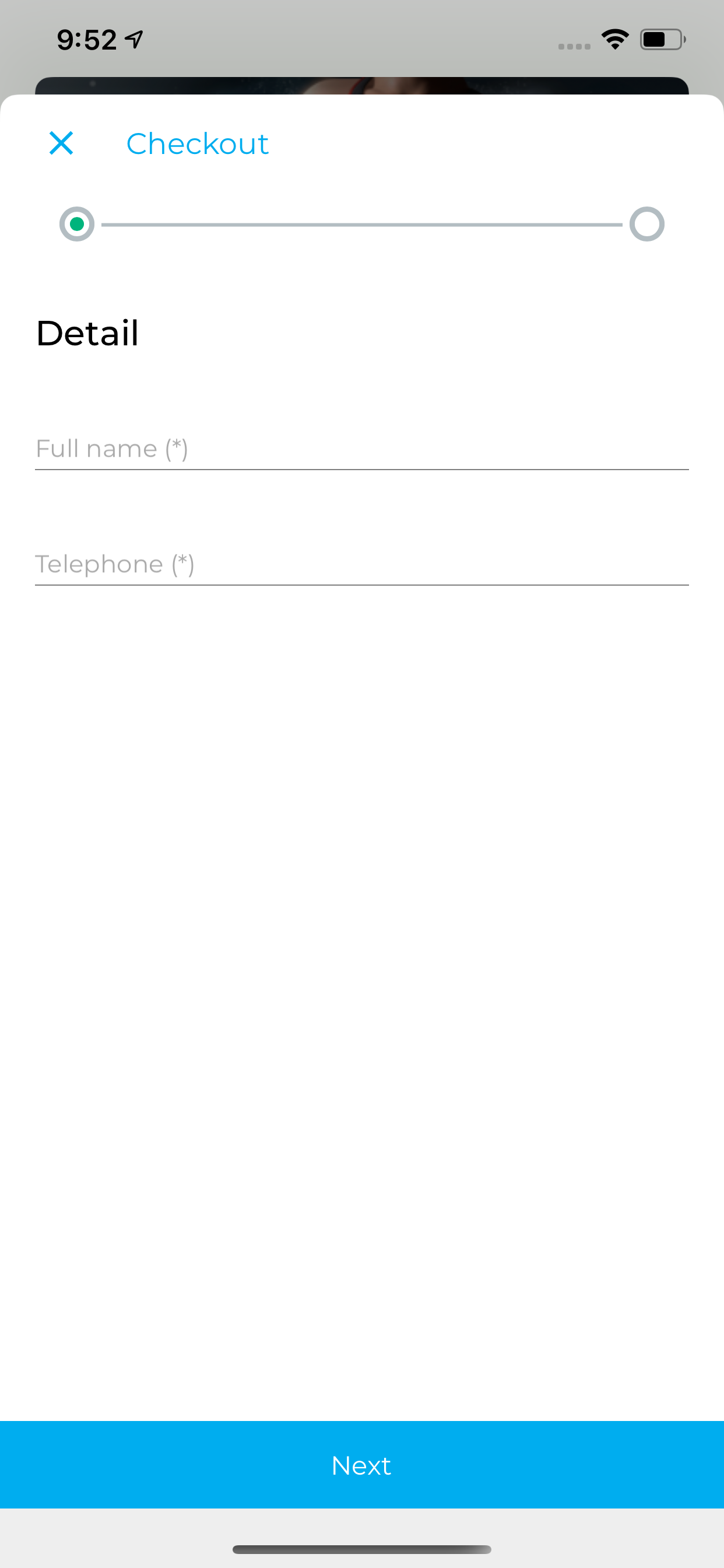**Image Caption:**

A smartphone screen displaying a form interface with various elements. At the top, the title is in grey text but incorrectly reads "9.2". The screen shows full wifi connectivity and displays some prompt or command that states "not feel better, check out".

Below the title, the form requires personal details including "Full Name" and "Telephone", both marked with an asterisk indicating mandatory fields. The location services icon is visible, indicating that these services are enabled on the smartphone.

The interface has a blue rectangle button labeled "Next" towards the bottom. The bottom part of the screen is grey, separated by a thin black line. The background of the screen interface is white with some underlying blue elements. There is a small black rectangle visible, suggesting another app or window might be layered beneath the current one.